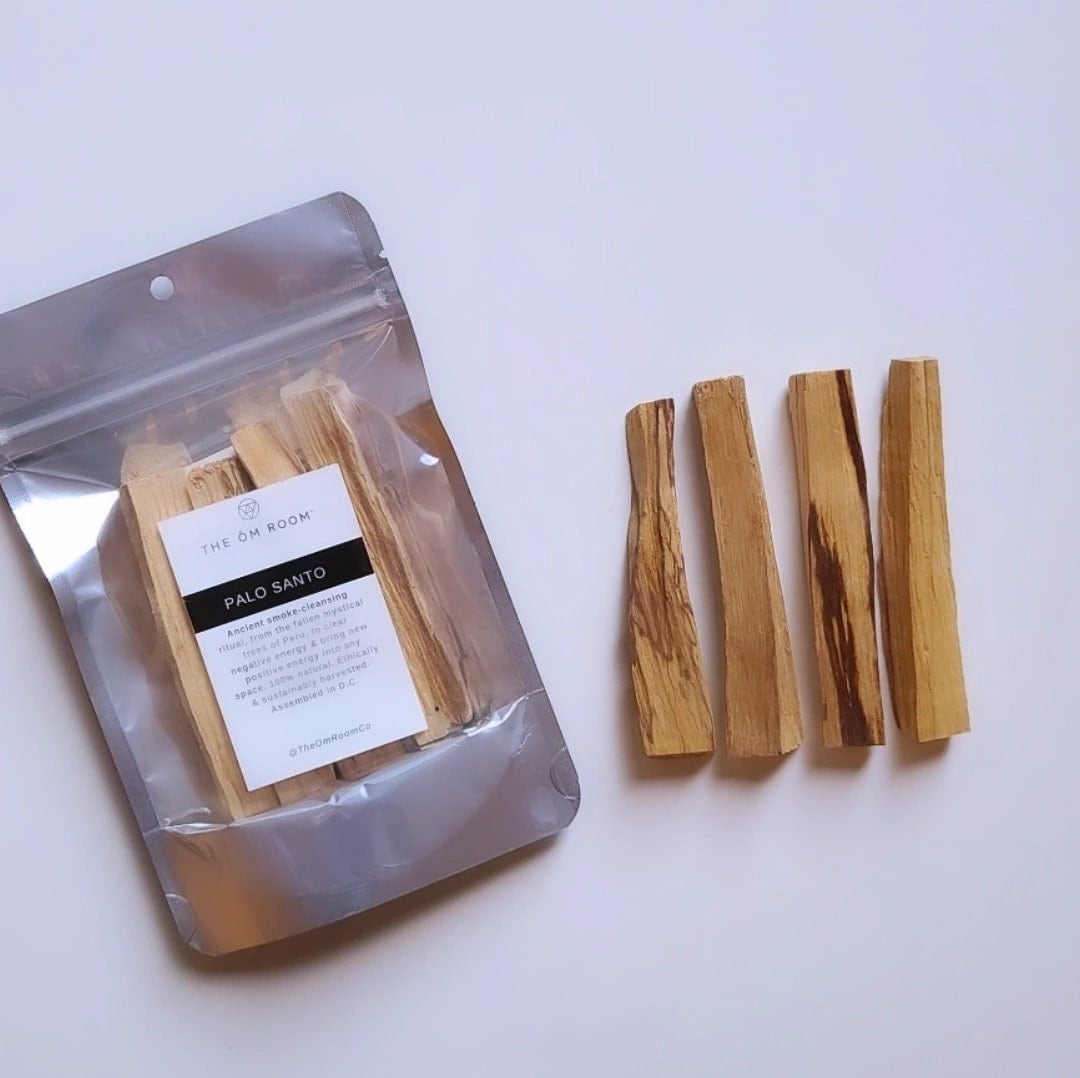This is a full-color, vertically oriented photograph taken indoors under artificial light. The background is a blend of light purple, lavender, and pinkish hues. Dominating the left side of the image is a purple cellophane package with a transparent section in the center, allowing a clear view of its contents—several small, brown wooden sticks, roughly 1.5 to 2 inches in length. The package has a white label affixed to its top, with "the OM room" written in dark letters, and below it, "Palo Santo" printed in white against a black band.

Adjacent to the package on the right, there are four similar wooden slivers, neatly arranged in a vertical stack. Each piece appears to vary slightly in shade, with one having distinctly darker wood at its base. The overall scene is minimalistic and centered around the mysterious wooden sticks with no further objects or text visible in the frame.